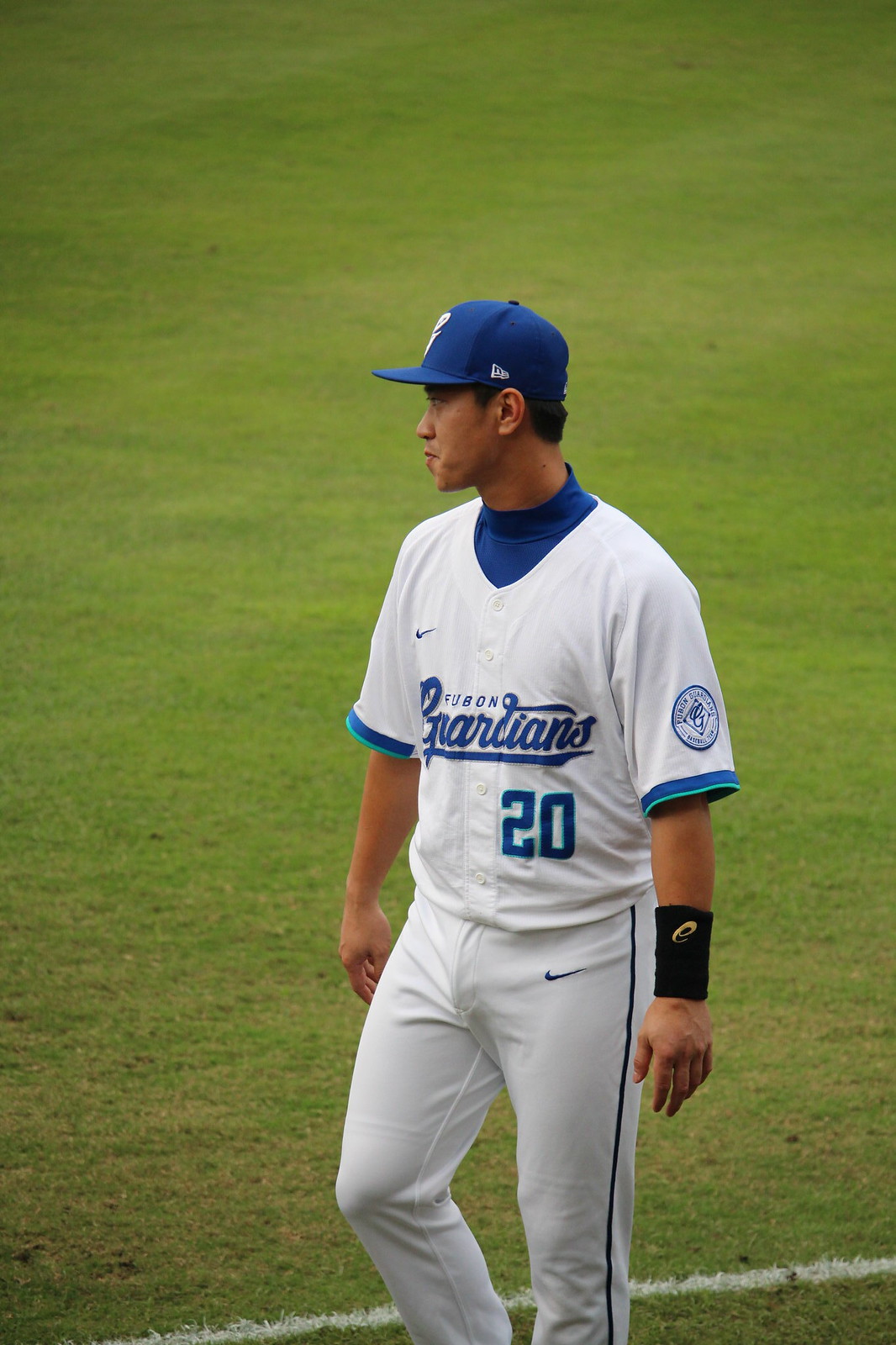The image depicts an Asian professional baseball player on a green field, captured facing forward but with his head turned to the left, showcasing his focused expression. He has black hair, tan skin, and is wearing a dark blue baseball cap adorned with white markings. The player is dressed in a white jersey with "Guardians" written in italic, handwritten-style blue text across the front, and "Fubon" above it. The jersey features a blue Nike swoosh on the left chest and the number 20 in blue below the Guardians text, outlined lightly. Both sleeves end with a blue and thin green stripe and the left sleeve includes a circular blue patch bearing the Fubon Guardians logo. Underneath his jersey, he sports a blue turtleneck undershirt and a black wristband with a yellow "E". His white pants, which have a thin blue stripe down the left leg, also display a blue Nike logo on the upper right section. The background features green grass with a lighter green hue and a white baseline running across the bottom right corner of the frame.